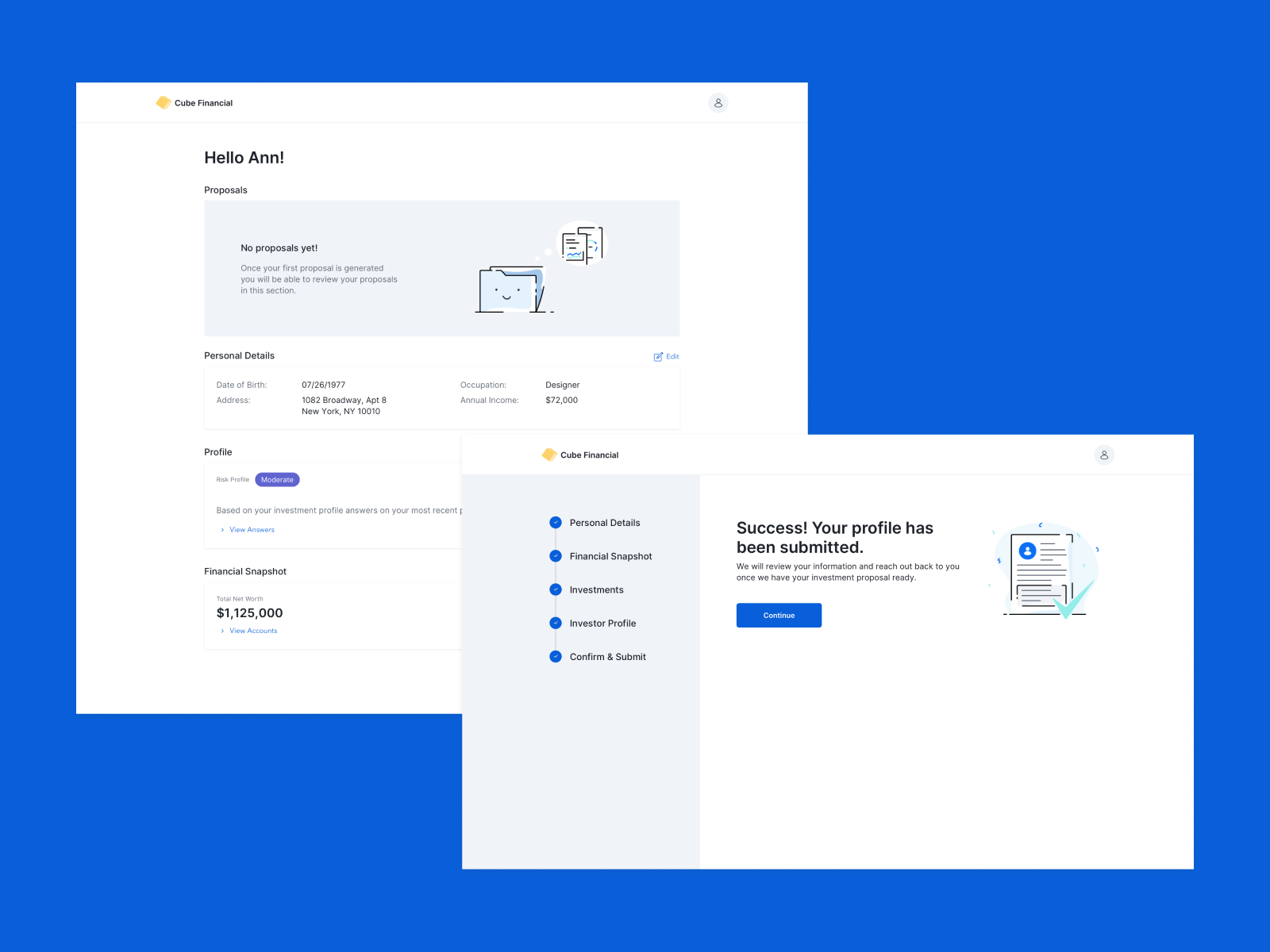Screen capture from the Cube Financial webpage displaying a mixed interface of background and an overlay pop-up window. On the left in the background, the main page features a header that warmly greets the user with "Hello Ann." Below this, it shows a section labeled "Proposals," which currently has no proposals listed. Following this, the user's personal details are visible, including their date of birth, address, occupation, and annual income. Further down, there's an option labeled "Profile," and beneath that, a section titled "Financial Snapshot," which reveals the individual’s financial standing at $1,125,000.

Shifting focus to the overlay in the lower right, this pop-up window reiterates the "Cube Financial" branding and features a vertical navigation column on the left, marked by blue dots. The column lists different sections: "Personal Details," "Financial Snapshot," "Investments," "Investor Profile," and "Confirm and Submit." 

To the right of this column, the content within the pop-up proudly announces "Success!" confirming that the user's profile has been successfully submitted. Additionally, there’s a "Continue" button accompanied by an icon depicting a chart with a blue check mark, symbolizing successful completion. This scene indicates that the user has finalized their profile setup process on the Cube Financial platform.